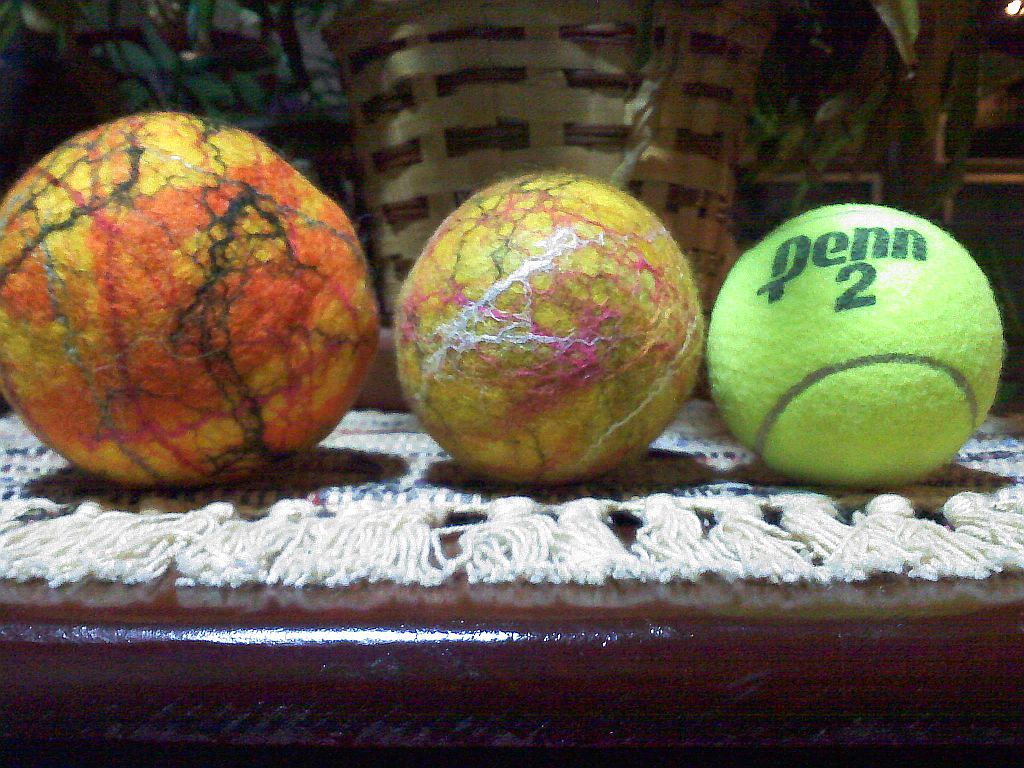This photograph showcases a detailed arrangement placed on a dark wooden surface, possibly a chest of drawers. On the wooden surface lies a white wool runner, interspersed with blue threads, resembling a small woven mat or carpet with frayed edges. At the forefront of the image, three distinct balls are positioned from left to right. 

The ball on the far left is the largest, about the size of a grapefruit. It is yellow with intricate, abstract patterns in orange, black, and red, resembling waves or neural pathways. The middle ball is slightly smaller, approximately the size of a baseball, and is yellow with threads of pink, white, and black interwoven throughout its surface. The ball on the right is a standard neon green tennis ball, marked with “Penn 2,” indicative of its brand. 

In the background, a large woven basket can be seen, partially obscured by leaves, which suggests the presence of some greenery or possibly a potted plant. The basket is constructed from wide and narrow wooden laths, adding to the rustic charm of the scene. This image offers a carefully composed view that merges natural textures and vibrant colors within a household setting.